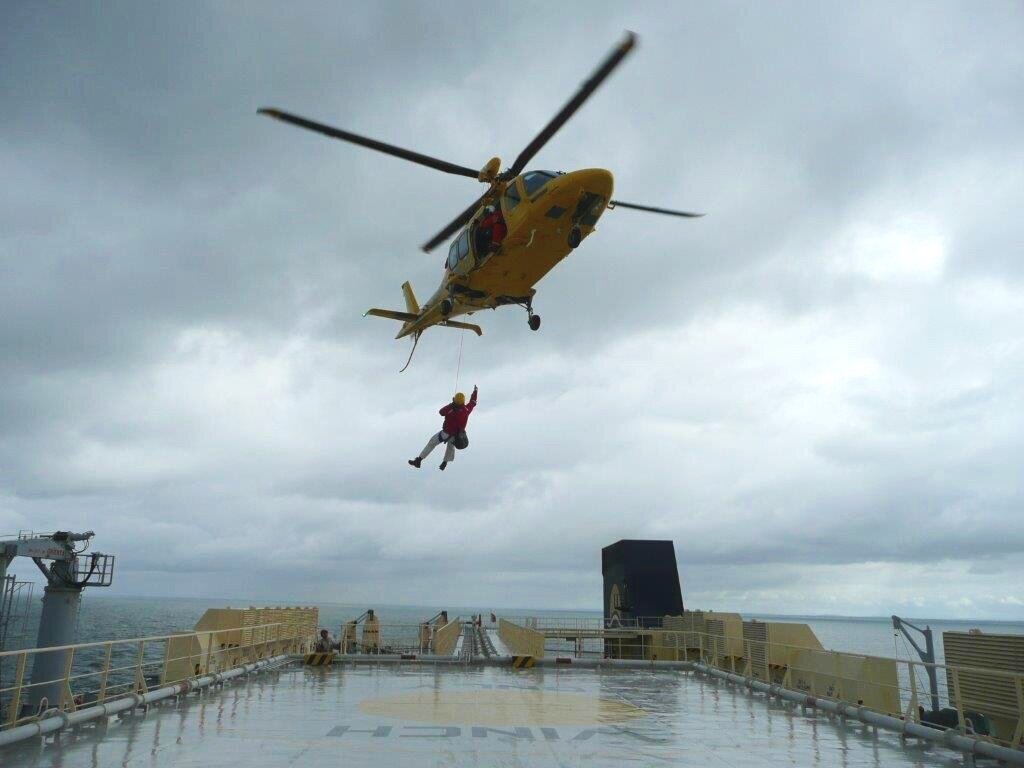A vibrant scene unfolds in this dynamic photograph of a yellow helicopter hovering mid-air against a backdrop of a blue and white sky, tinged with dark stormy clouds. The helicopter, prominently positioned towards the top center of the image, features four long blades spinning above. An individual clad in an orange suit is seen at the side door of the helicopter, seemingly overseeing an operation.

Suspended by a tether from the helicopter is another man, dressed in a red jacket and white pants, carrying a satchel on his back. His right arm is lifted, possibly reaching towards the helicopter, and he appears to be gazing upwards at it. Below them lies the shiny, gray deck of a large ship, likely an aircraft carrier, with beige-colored railings bordering its edges. Painted onto the deck are the word "WINCH" and what might be a hexagonal yellow logo.

The bottom part of the image reveals the vast expanse of water surrounding the ship, giving a clear indication that the scene takes place at sea. This photograph captures the intense moment of an air-to-ship rescue or operation amidst dramatic weather conditions.